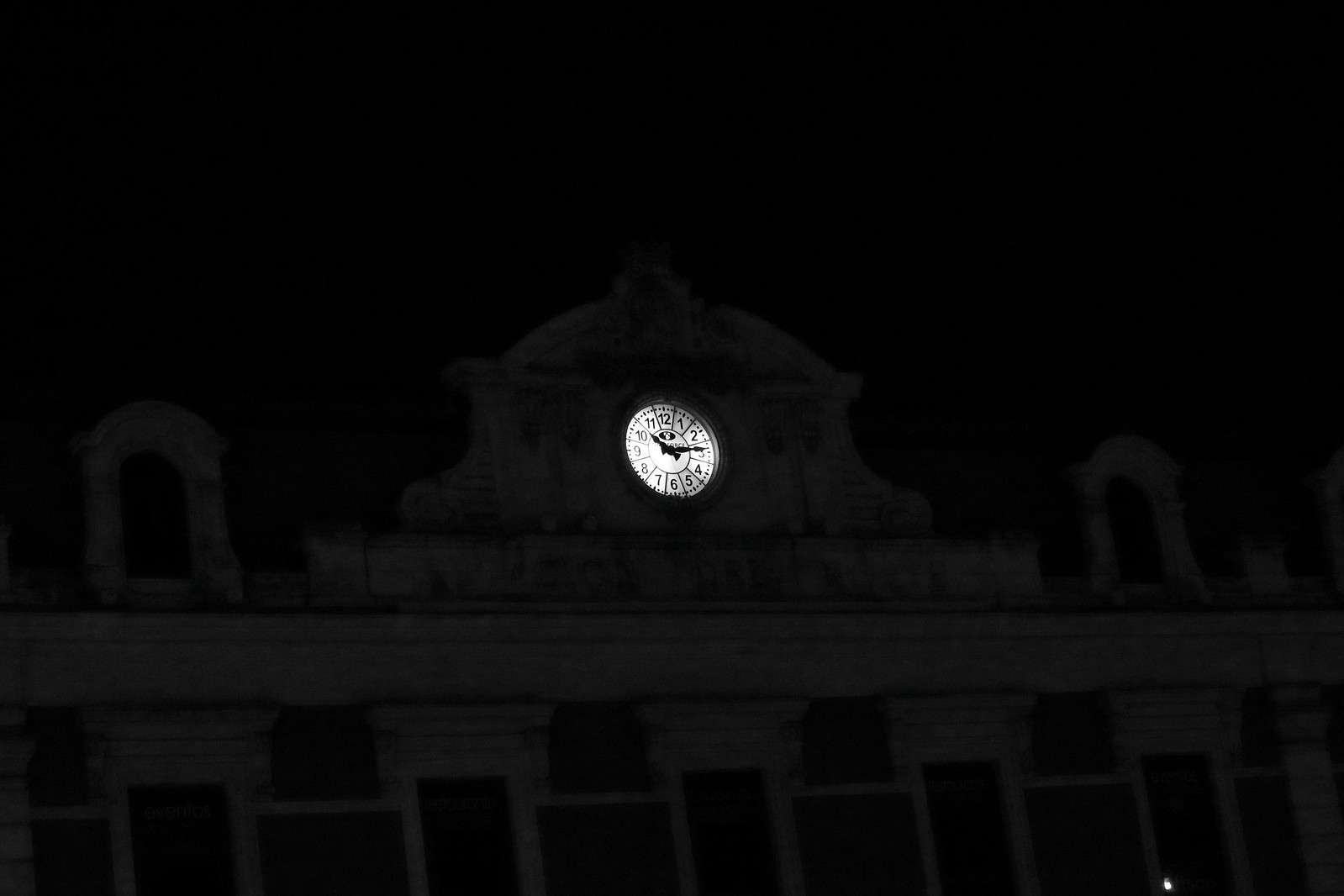A stately building, constructed from gray bricks, stands prominently against the night sky. The structure is accentuated by numerous towering pillars, adding to its majestic appearance. At the top of the building, two shorter pillars rise elegantly. Dominating the center is an ornate semi-circular design, within which rests a beautifully illuminated clock. The clock's face is clearly visible, displaying the numbers 1 through 12 in black, accompanied by intricately designed black minute and hour hands with swirled patterns at the top, tapering into straighter lines at the bottom. The clock shows the time as 10:14.